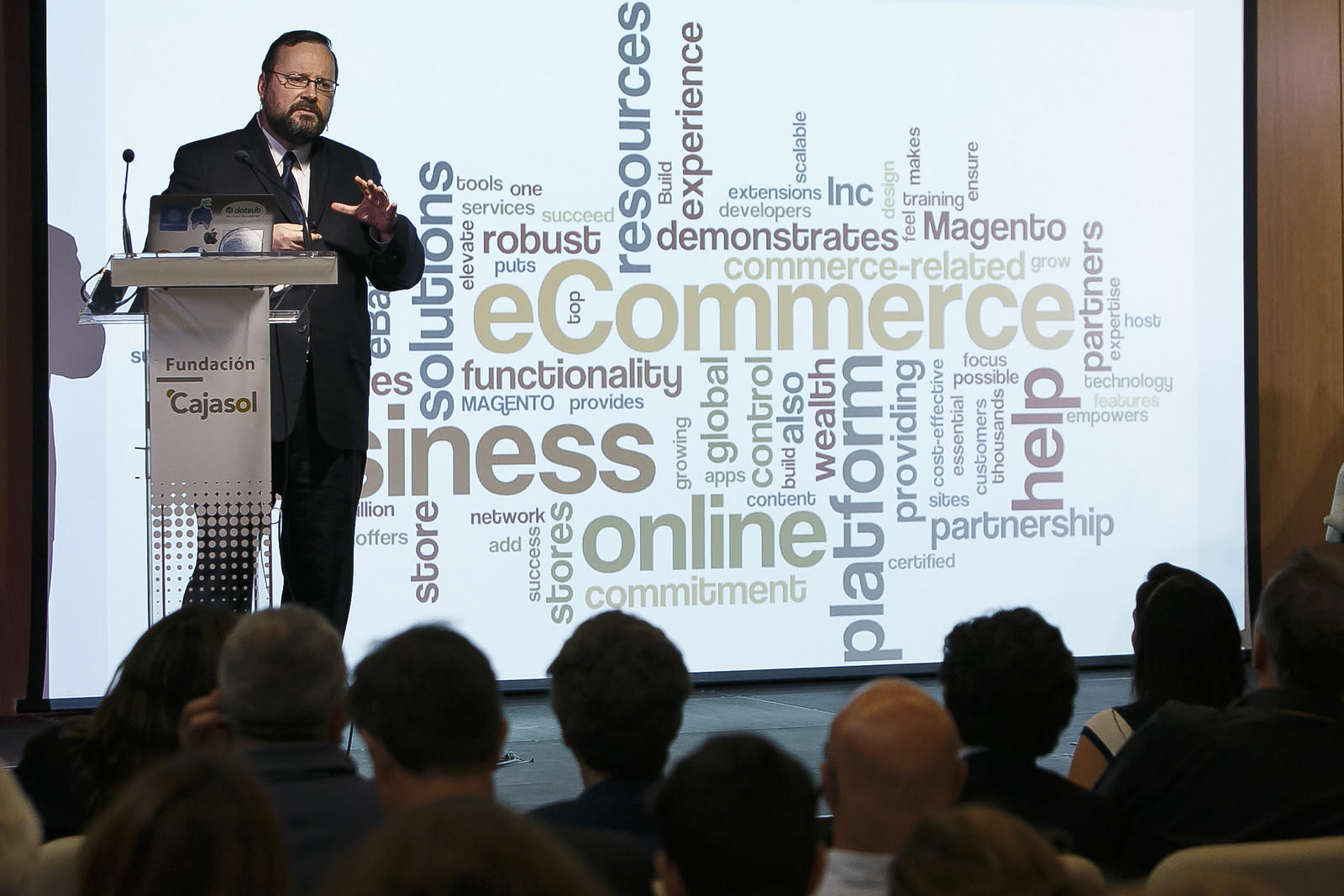In this indoor photograph, we see a man standing at a glass podium on the left side of a stage, addressing an audience. He is of Caucasian descent, with short brown hair, a beard, mustache, and glasses, wearing a black business suit paired with a black tie and a white collared shirt. His hand is extended as he speaks, emphasizing his points. The podium bears a banner that reads "Fundación Cajasol." Behind him, a white backdrop or screen displays various words in different colors and orientations, including phrases like "e-commerce," "business," "online," "demonstrates," "Magneto," "robust," "store," "solutions," "platform," "resources," "experience," "global," "control," and "wealth." The audience, of which we can see the first three rows of heads, listens attentively to his presentation.